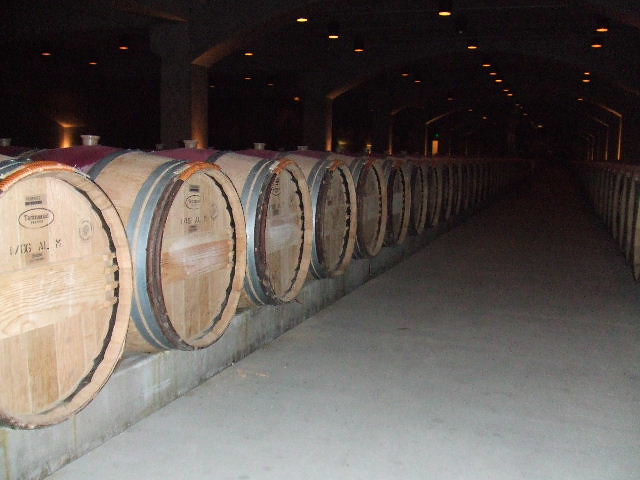The photograph captures a dimly lit, rectangular room within a dark brown warehouse resembling a winery or distillery. It prominently features rows of large, light tan wooden barrels with teal midsections and silver metallic bands, which are stacked on raised concrete platforms. These barrels are arranged on their sides and aligned along a narrow gray concrete aisle that appears to slightly veer rightward, creating a diagonal visual effect. The barrels stretch from the bottom left corner of the image towards the middle, disappearing into the dimly lit background where evenly spaced circular lights, casting faint yellowish or orangey glows, hang overhead. The barrels bear black text and logos, mostly illegible, likely indicating dates or serial numbers. The entire scene is illuminated primarily by the camera's flash, highlighting the first few barrels with additional copper tops reflecting the ambient light. The image is devoid of people, animals, plants, or motorized vehicles, focusing solely on the barrels within the austere, cavernous space.